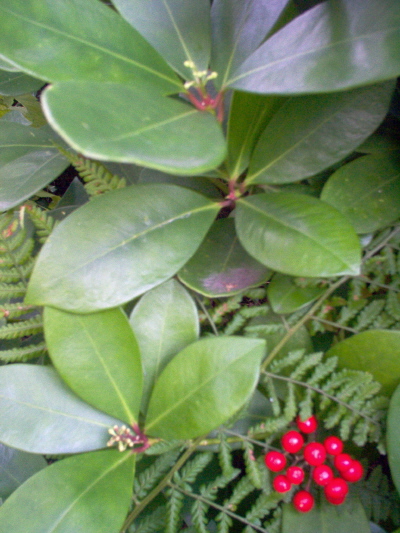This vivid, full-color outdoor photograph captures a multitude of small plants with delicate leaves and slender stems. The greenery is lush and vibrant, set against a backdrop of ample natural daylight that illuminates every detail. In the bottom right-hand corner of the image, clusters of red berries can be seen, although the exact type is indiscernible as this portion of the image is slightly blurred. The rest of the image remains in sharp focus, showcasing a rich palette of greens and reds. The scene is serene and untouched by human presence, with no people, vehicles, animals, or text, highlighting the beauty of nature in its purest form.